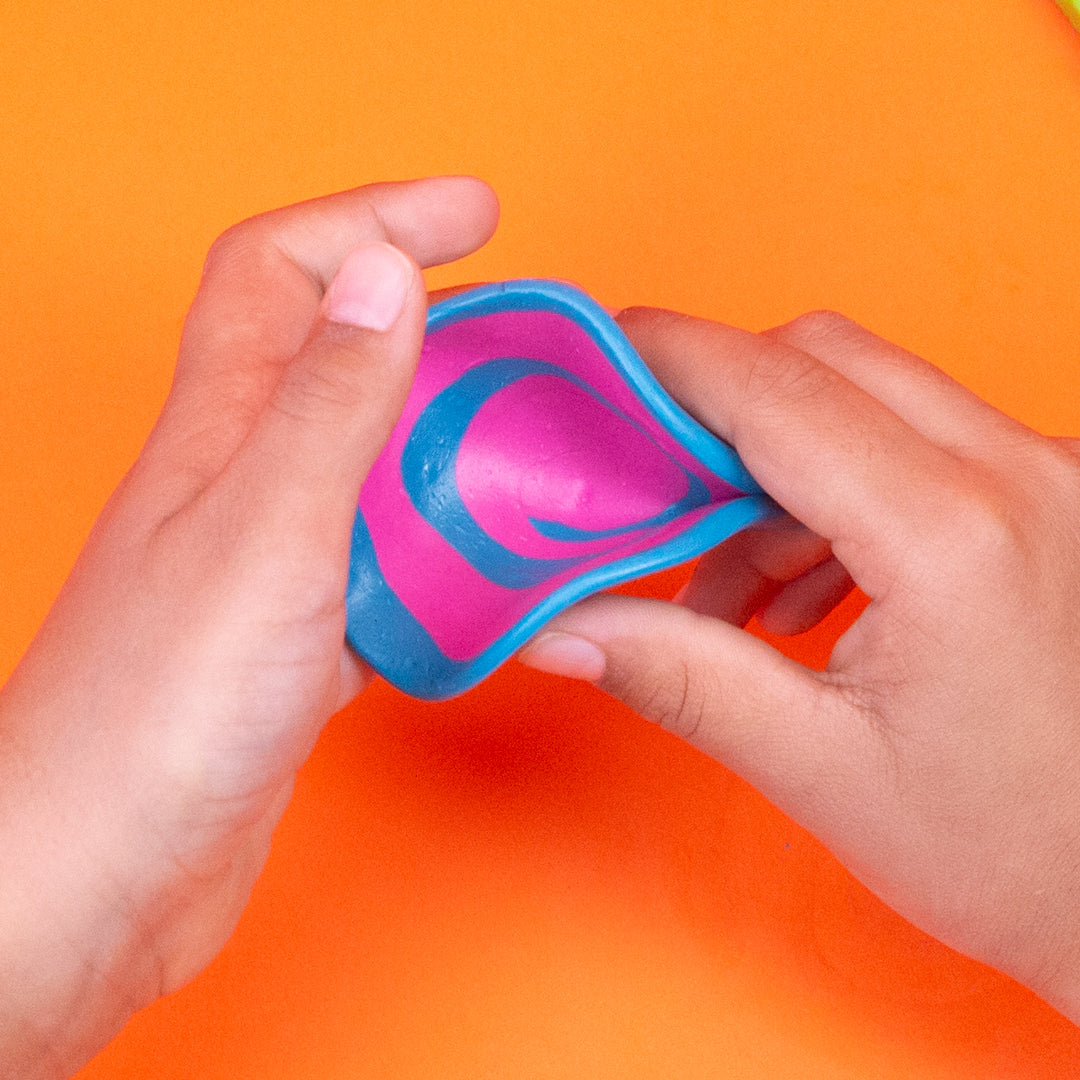The image features two hands pressing and molding a spherical object that appears to be made of a soft, pliable material, reminiscent of putty or Play-Doh. The object is predominantly pink with blue swirls and a blue outer edge, crinkled and indented where the thumbs and fingers exert pressure. The object has a bowl-like shape with the edges pushed up and the center depressed. The background is a vivid orange, transitioning to a darker, redder shade directly beneath the object, with hints of yellow surrounding it. The hands are centrally positioned, one on the left and one on the right, and are relatively hairless with normal-sized fingers. The hands likely belong to a white person, though this detail is not certain.